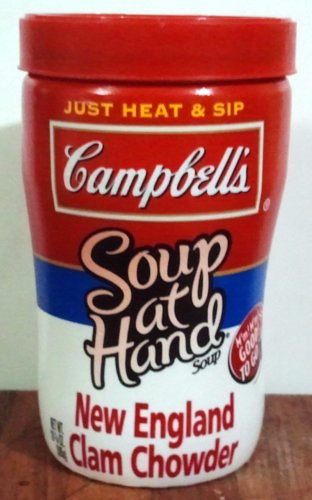A small, individual-sized container of Campbell's Soup at Hand sits on a medium-toned wooden surface against a plain white wall. The cup is designed with a red top section, a blue strip around the middle, and a white bottom section. It features a red plastic screw-on lid. The label prominently displays the instructions "Just Heat and Sip" and the iconic "Campbell's" logo across the red, blue, and white sections. Towards the bottom of the label, it reads "New England Clam Chowder." To the side, there is a round emblem with the phrase "Mmm... Good to Go."